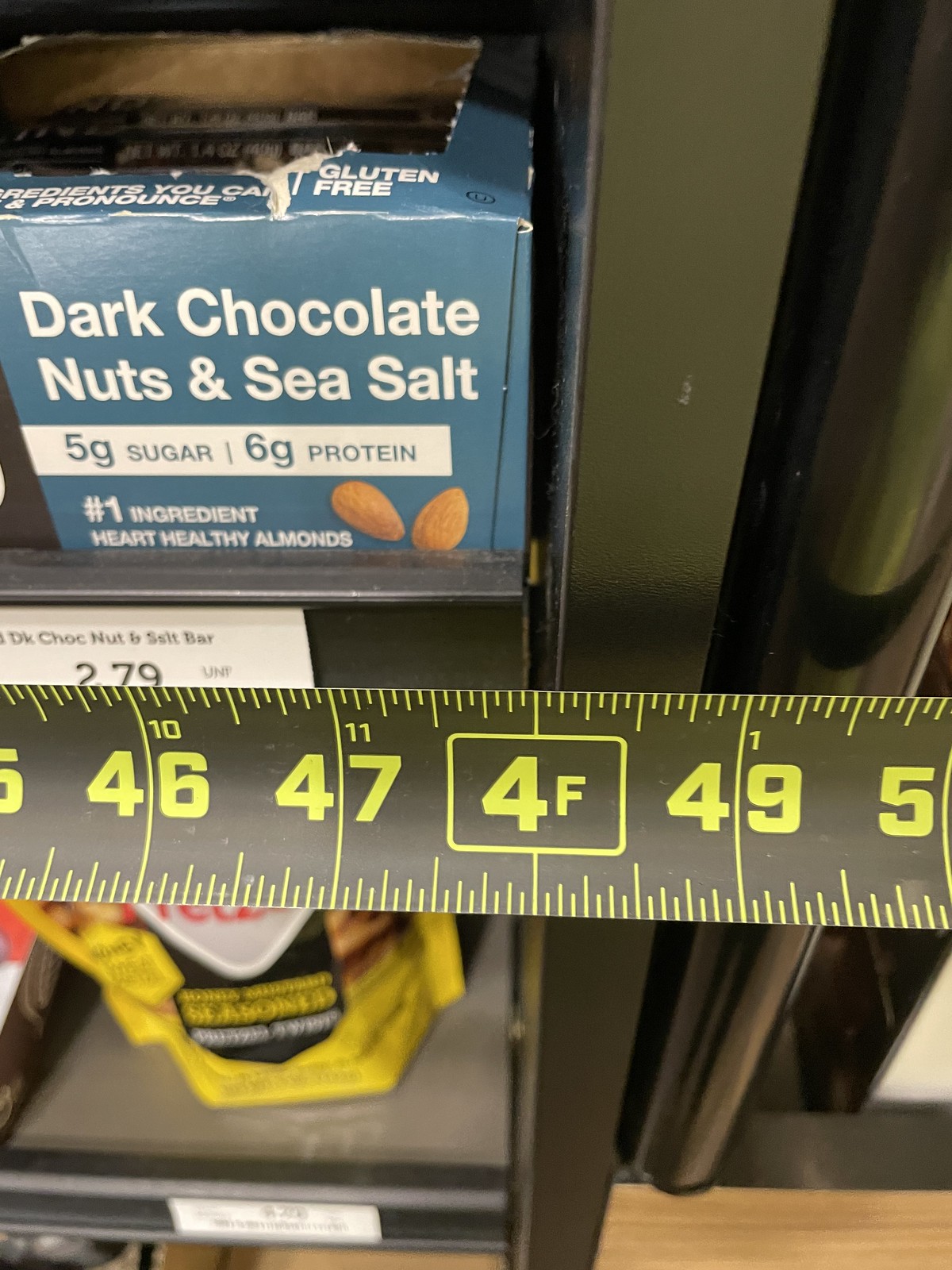In this detailed photograph, a measuring tape prominently spans horizontally across the middle of the frame, providing an accurate measurement of exactly 4 feet to the edge of the shelf. The measuring tape itself is black with yellow markings, giving a clear contrast that enhances readability. Positioned to the left of the image is a tall, metal shelving unit. On one of the shelves near the top, there is an open blue square box containing performance bars. The box is detailed with text indicating that the bars are flavored with dark chocolate, nuts, and sea salt, boasting 5 grams of sugar and 6 grams of protein, with heart-healthy almonds as the primary ingredient. To the right of the image, the rounded edge of what appears to be a beverage cooler is partially visible, adding context to the setting of the scene.